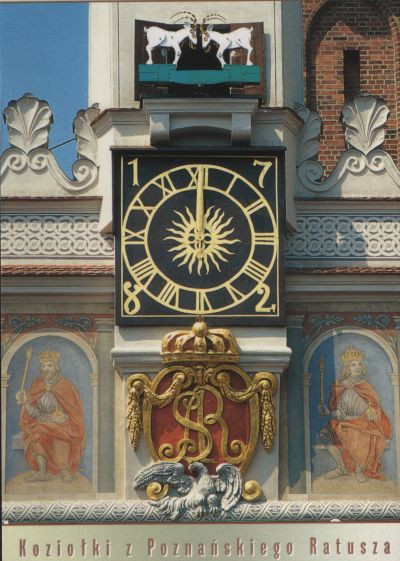The photograph captures an elaborate architectural detail of a European building, prominently featuring a large, ornate clock. The clock is framed in a square, black bezel with a round face set within it, showcasing elegant golden Roman numerals from I to XII and a sunburst motif in the center. Each corner of the square frame displays a numeral: 1 in the upper left, 7 in the upper right, 2 in the lower right, and 8 in the lower left. 

Above the clock, two white rams, seemingly made of wood or stone, face each other as if in mid-charge. The background consists of intricate white brickwork decorated with leaf-like patterns. Flanking the clock on either side are frescoes depicting royal figures adorned in red robes and holding scepters, likely representing knights or kings. 

Below the clock lies a grand red and gold crest with elaborate designs, crowned and featuring an eagle-like figure in silver beneath it. At the bottom of the image, an inscription in a European language reads "Kozlodki Poznanskiego Ratusa," hinting at a Polish origin. The intricate details and the architectural style strongly suggest a heritage building, possibly in a historic European city center.